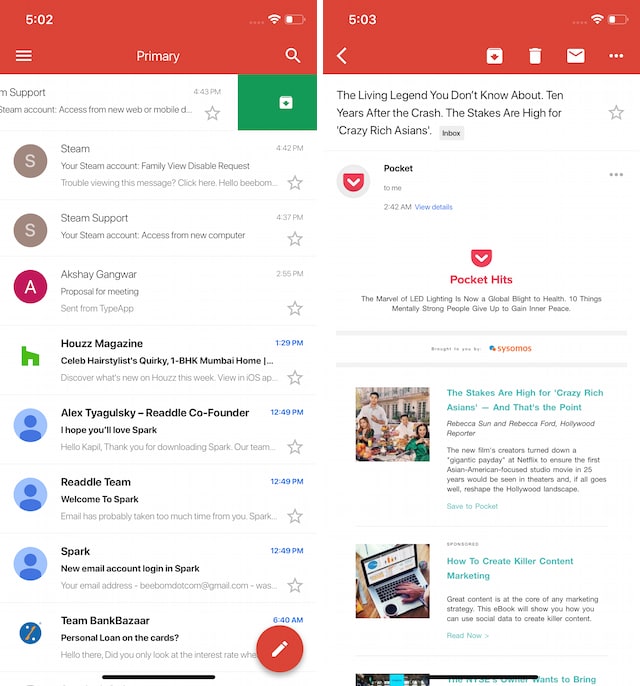**Descriptive Caption:**

"Two images of mobile screens are displayed side by side under the theme of websites. The image on the left shows a phone screen with the text '502' prominently displayed along with 'Primary' and 'Support'. It includes a list featuring 'Steam', 'Your Steam Account', 'Family View', 'Steam Support', followed by names such as 'Akshay Gangar', 'Howe Magazine', 'Alex Riedel, co-founder', and 'Riedel Team'. There is also a mention of 'Welcome to Spark', with options to 'Log in to Spark' for a 'New email account', and information regarding 'Team Bank Bazaar' suggesting a 'Personal loan on the cards'.

The second image highlights a different phone screen featuring icons for 'Download', 'Trash', and 'Email' at the bottom. The top of the screen is headlined with various articles including 'A Living Legend You Don't Know About', '10 Years After the Crash', 'Stakes are High for Crazy Rich Asians', and categories like 'Pocket and Pocket Hits' along with 'How to Create Killer Content' and 'Marketing'."